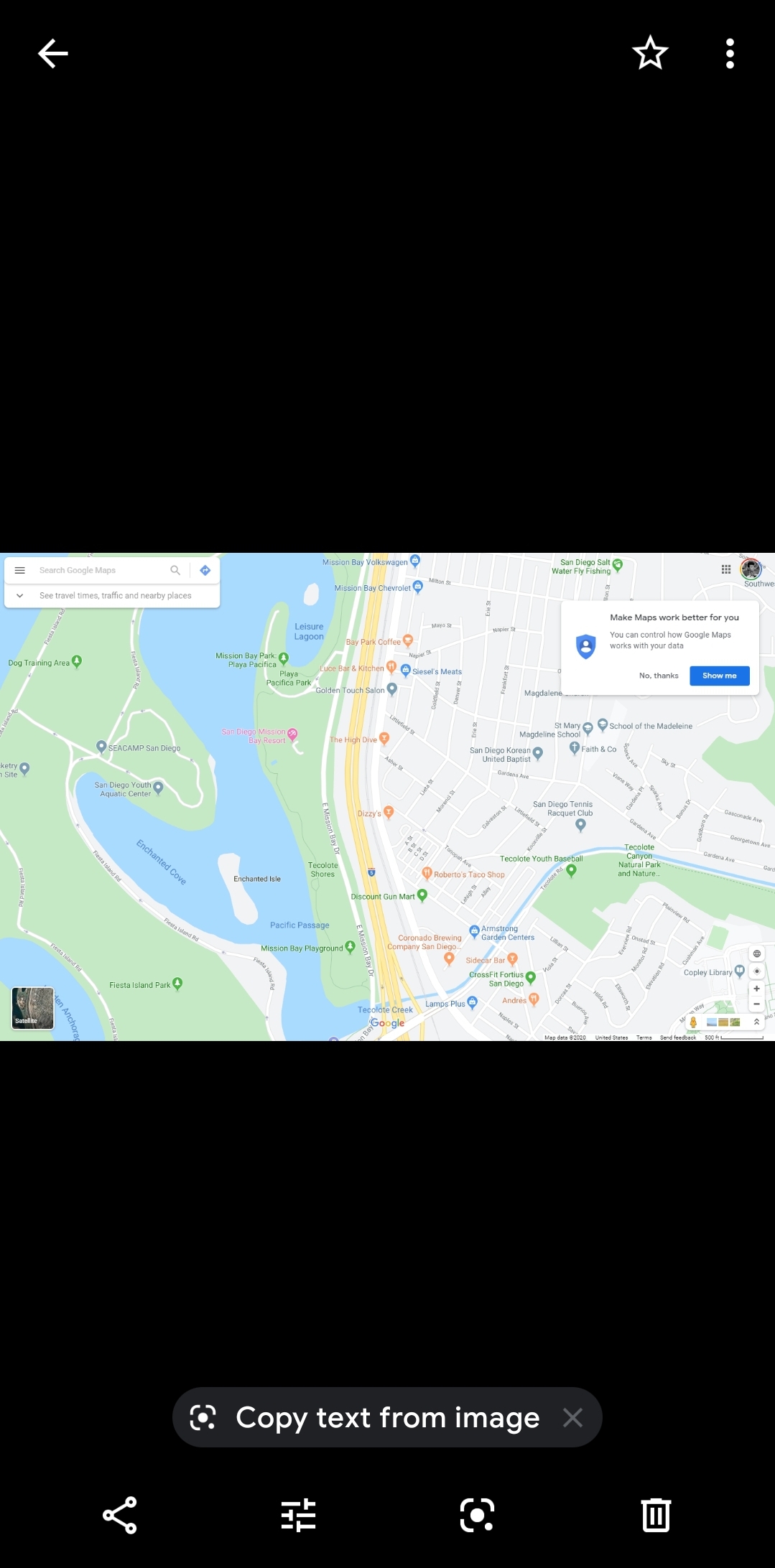This detailed map vividly illustrates various regions and features. Predominantly green areas represent dense forested zones, while a distinct blue section highlights a body of water. On the opposite side, a bustling cityscape is depicted, complete with several noted landmarks and destinations. To the right of this urban area, a small green patch suggests additional greenery, juxtaposed against another smaller section of the city accompanied by an extra patch of green. Overlaid on the map is a question box, presumably containing informational content. On the left side, there's a enigmatic posting contrasted against a black background, adorned with a scattering of dots and a prominently positioned star.